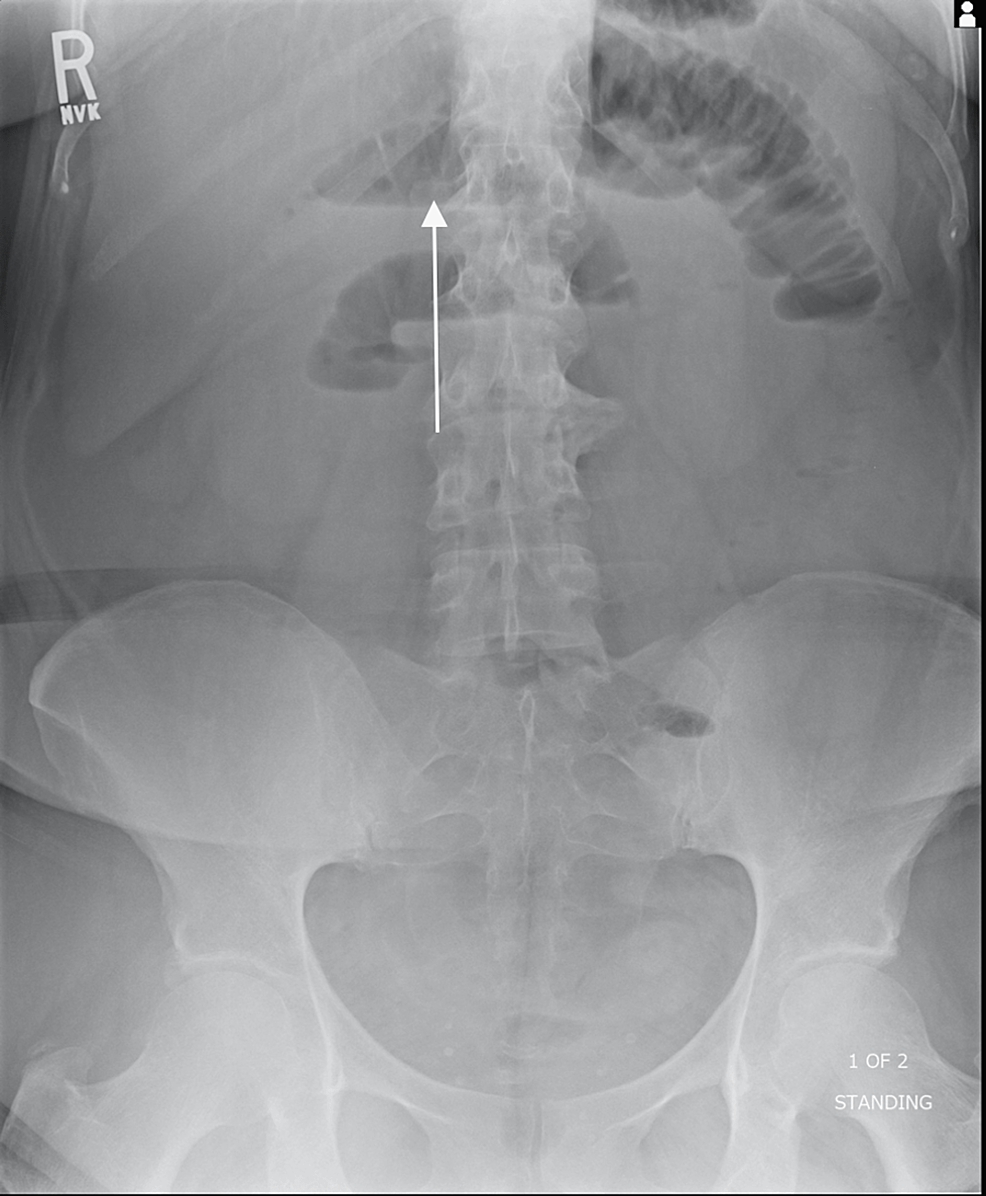The vertical X-ray image captures the pelvic region and lower back, highlighting the pelvis, hip bones, and the lower vertebrae with a slight curve to the right at a 5-degree angle. Dominated by varying shades of white and grey, the image features several overlays: in the top right, a black square with a white head-and-shoulders icon is positioned next to bold text reading 'R' and smaller letters 'NVK.' In the bottom right, finer text notes "1 of 2" and "standing." A thin, one-inch high white arrow, located to the left of the spine, points upwards towards a small, darker area near the vertebrae, possibly indicating a mass or ruptured disc. In the background, portions of the rib cage are visible extending upwards beyond the main focus area.